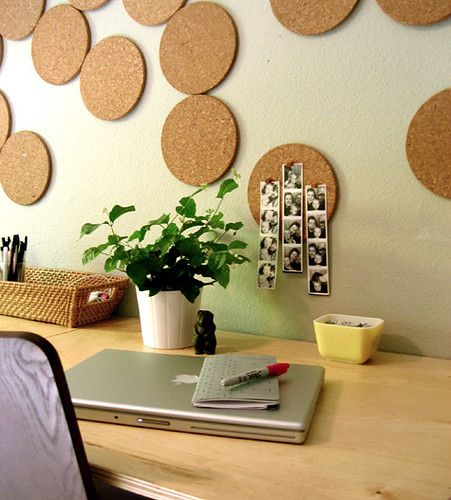This color photograph, taken during the daytime with natural light coming from the left, captures a detailed view of a workspace featuring a light oak-colored wooden desk. On the desk sits a closed silver Apple laptop with a planner on top and a red Sharpie marker placed nearby. Behind the laptop is a white flower pot with a green plant that appears to have fake leaves. To the left of the plant, a brown wicker basket holds a glass filled with pencils and pens. The workspace also includes a small black figurine and a yellow pot, which adds a splash of color. The desk is accompanied by a wooden chair. On the wall above, large circular cork boards display strips of photographs pinned to them, including photo booth pictures of two people.